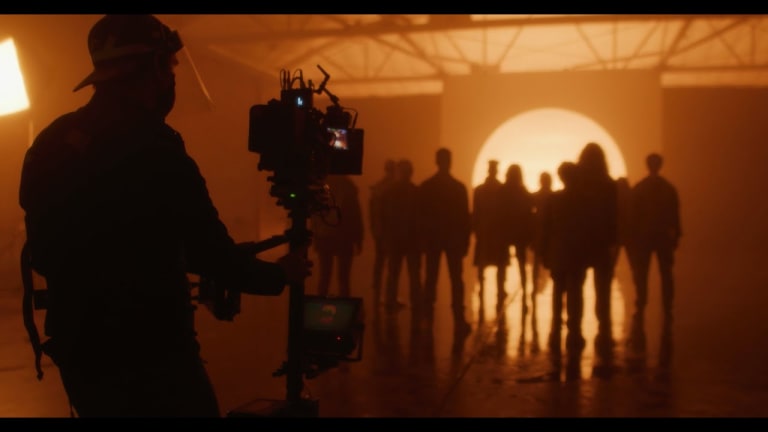This illustrative photograph showcases a silhouette-dominated scene bathed in an orange-brown hue. On the left side, a man in a backward cap, whose features are indiscernible, stands prominently holding a tall, elaborate movie camera directed to the right. Facing away from us, he captures a group of featureless, blurry silhouettes positioned towards the center and the right side of the image. Some members of the group appear close to each other, while others are more spaced out. They all seem to be gazing at a radiant, golden sphere reminiscent of the Sun. The scene, suggestive of a movie set, is draped in a blend of yellow and black tones, evoking a modern yet somewhat surreal aesthetic.